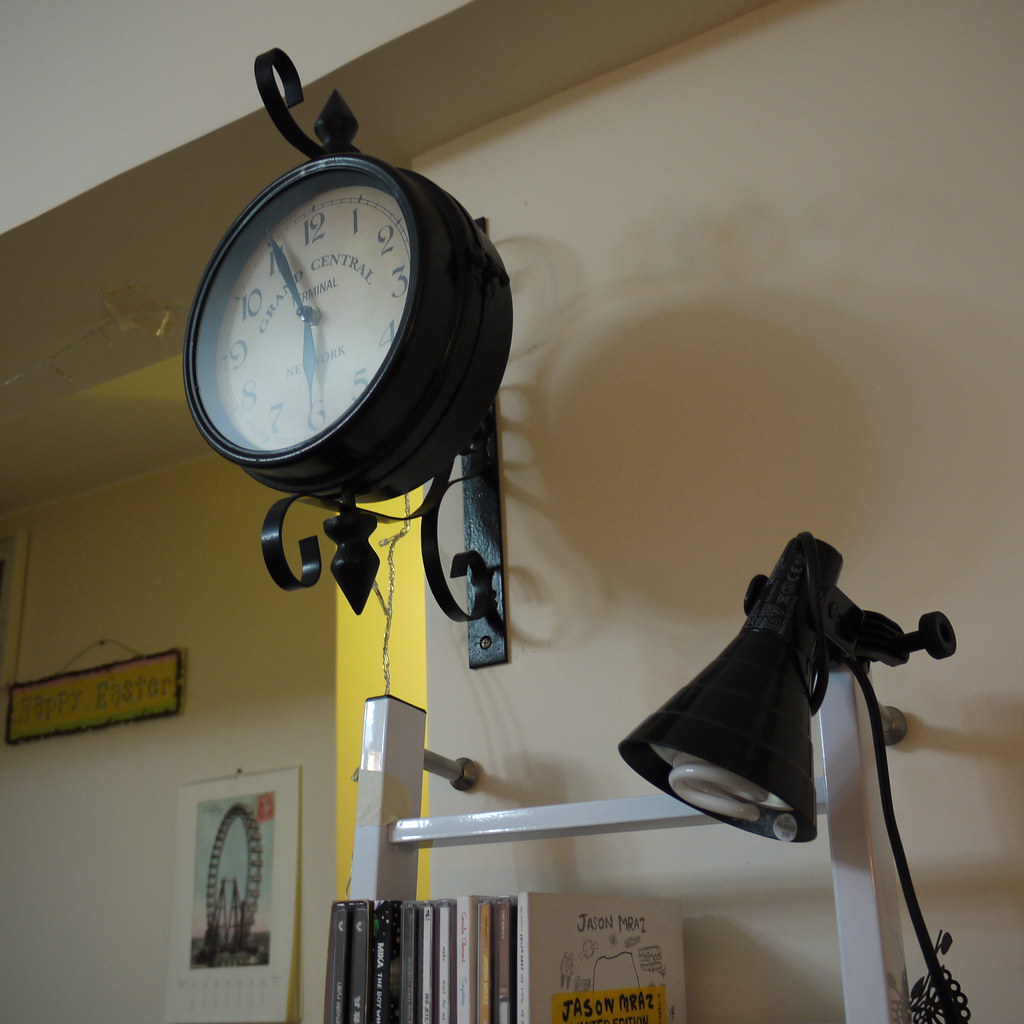The image depicts the interior of a room with a variety of elements. In the bottom right corner, a thin black line emerges, evolving into a black lampshade encasing a white, spirally light bulb. To the left of the lampshade, a white shelving unit is visible, displaying a series of books. Only the outer edges of the books are visible, except for the book on the far right. Above the shelving, a yellow strip runs along the wall, which is gray in color. Centrally placed on the wall is a black, circular clock with numbers marking each hour from 1 to 12. The clock's hands indicate that the time is 11:30. On the left-hand side of the image, a sign with a yellow background that reads "Happy Easter" adds a festive touch to the scene.